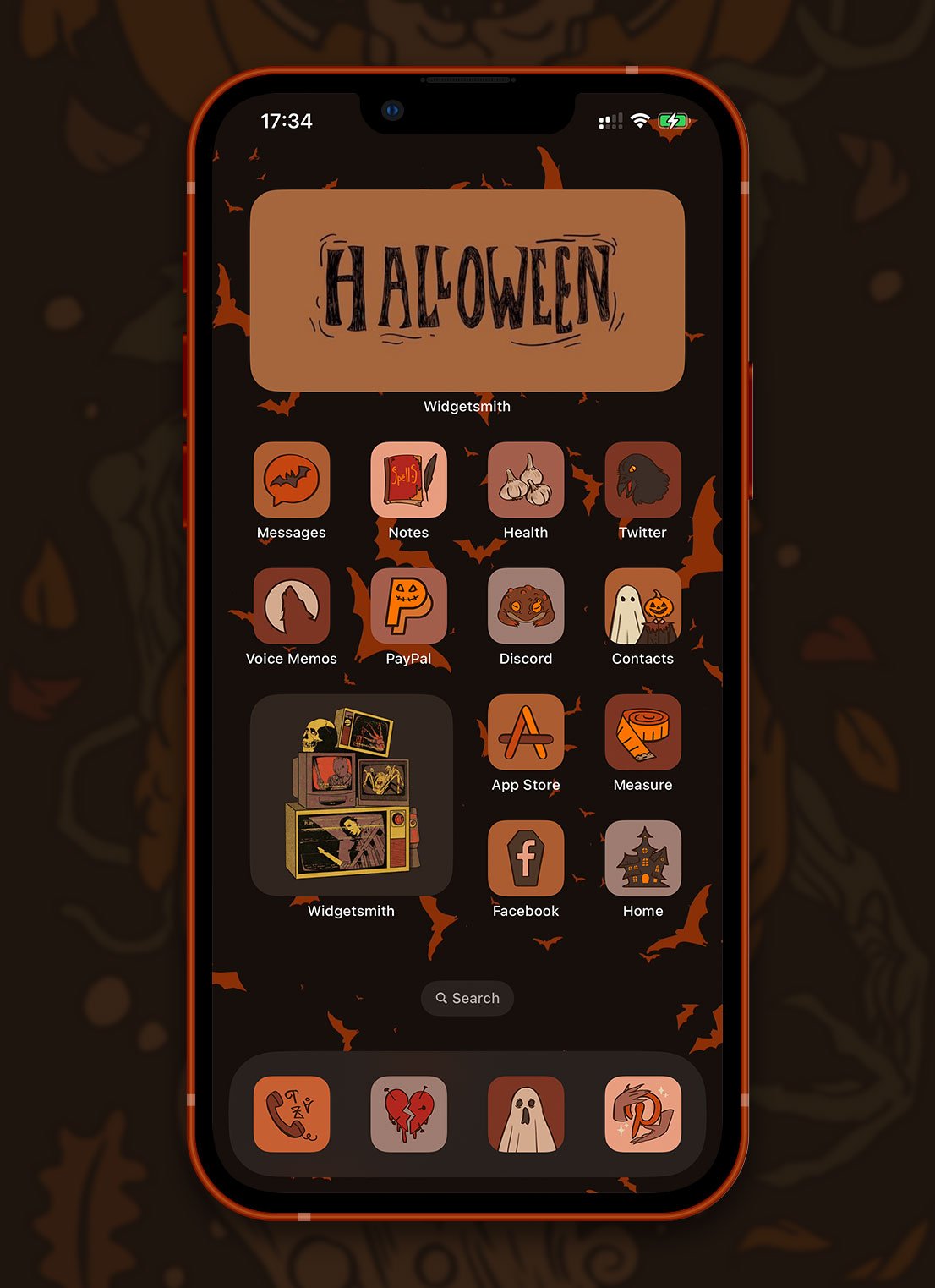In the image, the background is adorned with a tangle of branches, evoking a spookily atmospheric, Halloween-esque scene. Central to the image is a smartphone screen displaying a Halloween-themed home screen. The time is shown as 17:34, with the Wi-Fi signal and battery indicators present at the top right.

The smartphone features various Halloween-themed icons and widgets. The top left corner has a brown square widget labeled "Halloween" by Widget Smith, showing a stack of what appear to be televisions. The app icons include Messages, Notes (resembling a notebook), Twitter, and several others reimagined for Halloween. One icon portrays a black girl with the label "Voice Memo." There are also icons for PayPal, Discord (both in Halloween themes), Contacts (depicting a ghost and a pumpkin head), App Store, Measure, and Facebook. 

At the bottom, the home and search icons are visible, surrounded by Halloween decorations. The edges of the screen are distinctly orange, and bats can be seen flying around, enhancing the eerie Halloween ambiance. Other icons include a heart, a ghost, a clown, and what might be a headset, all contributing to the overall spooky effect of the smartphone display.